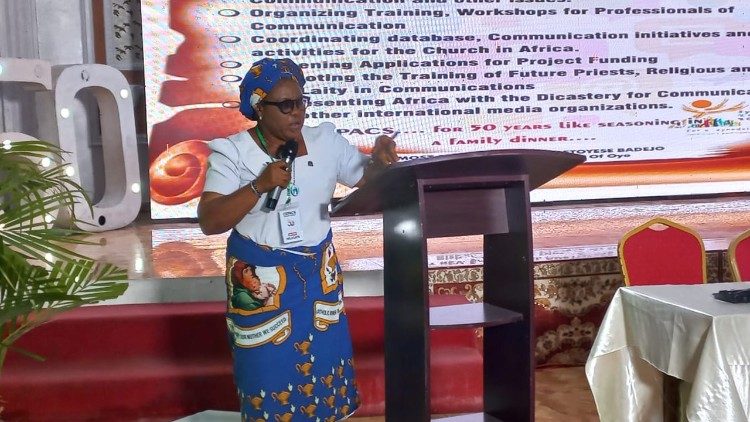In a landscape photograph, an African American woman stands on the floor, giving a presentation in front of a large, illuminated "50" sign on a stage. She wears a bright white short-sleeved blouse paired with a vibrant blue skirt adorned with intricate designs, including images of a mother holding a child and what appear to be genie lamps or teapot symbols. Completing her outfit is a blue head covering that matches her skirt. She holds a black microphone in her right hand, which has glasses perched on her nose, and she leans against a brown wooden podium, a green ribbon around her neck holding her credentials. 

In the background, a large projection screen displays bullet points detailing her discussion topics, such as "Organizing Training Workshops for Professionals of Communication" and "Coordinating Database Communication Initiatives and Activities for the Church in Africa," suggesting the presentation’s religious context. To her left, there is a table draped with a white silk tablecloth, flanked by empty red chairs, hinting at a formal event. The setting, accentuated by the celebratory “50” sign, implies a significant anniversary, possibly for a church or organization celebrating its 50th year milestone.